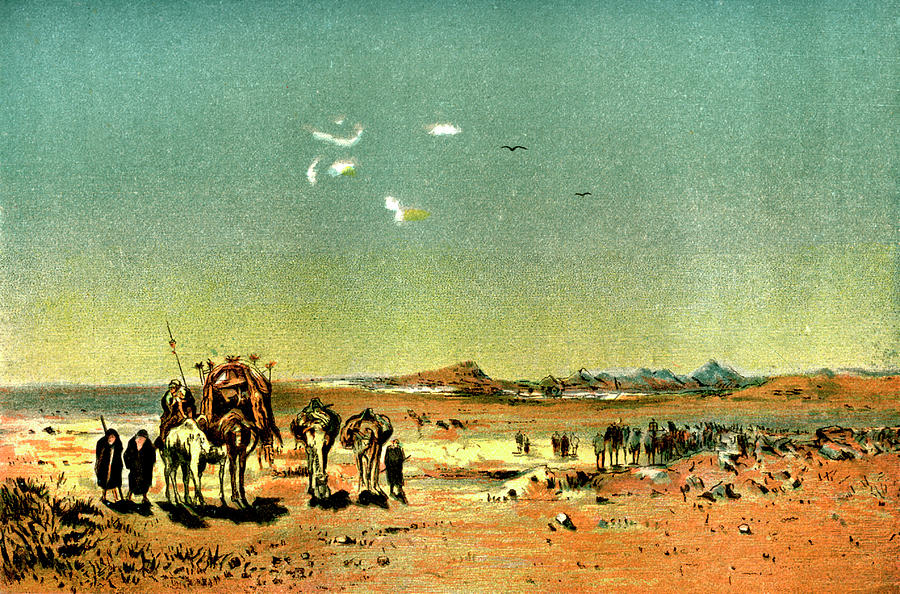The image is a rectangular, horizontal painting that exudes an ancient, historical aura. The scene seems to reflect a significant gathering or migratory activity, possibly a battle or a mass trek across a sandy expanse. The earth is predominantly brown, tan, and sandy with patches of white and hints of greenery, creating an almost desolate, desert-like impression.

On the left side of the painting, a horse-drawn carriage or stagecoach is visible, accompanied by a few camels carrying hefty loads, possibly transporting people. The camels and their handlers are detailed with long robes and staffs, suggestive of an age-old journey. There are a few animals and small, indistinct figures on the right, adding complexity to the ensemble, though they are less detailed and harder to discern.

Above, the sky transitions from rich blue to muted shades with scattered white clouds and two black birds. In the distance, a stretch of bluish-green water suggests a river or an ocean, bordered by low hills. The overall scene presents a stark yet vivid tableau of ancient travelers, moving as a caravan across a vast, arid landscape under a broad, enduring sky.